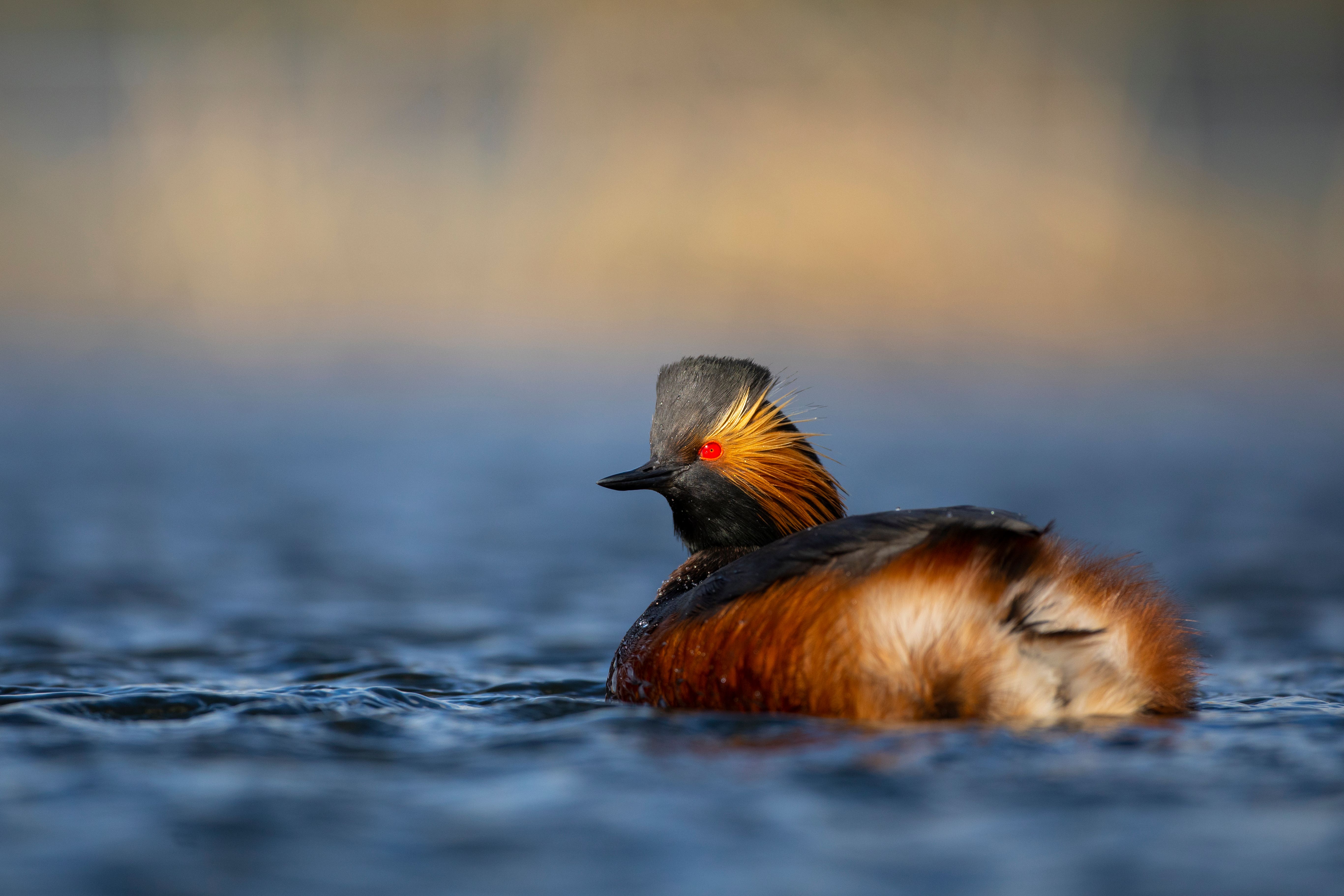This is a color photograph of a distinctive duck-like bird, swimming in a calm, blue lake. The bird is centered and in sharp focus, while the background and foreground are deliberately blurred, creating a soft, light yellow-brown backdrop. The bird is swimming away from the viewer, but its head is turned to the left, offering a clear side profile. It has a thin, black beak and a striking head adorned with tufted, grayish-charcoal feathers resembling a mohawk. Its eyes are a vivid red, with feathers extending from them that look like elongated eyelashes in light yellow and orange hues. The bird's neck and throat are black, its upper back features dark feathers, and its lower body is a mix of reddish-brown, black, and white, with its tail feathers being predominantly white. The water around the bird shows only a few gentle ripples, enhancing the tranquility of the scene.